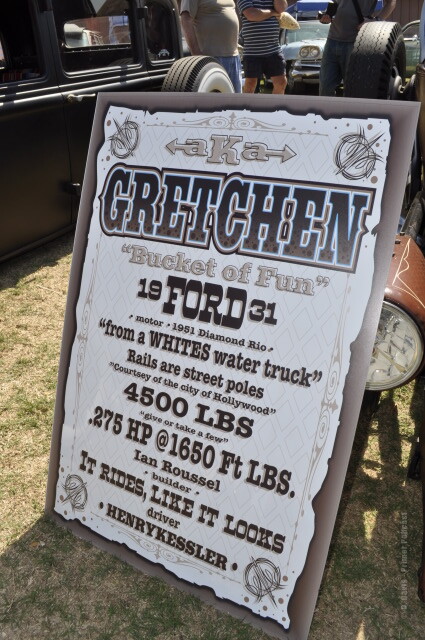The photograph captures an outdoor event featuring a vintage display sign prominently positioned on a patch of grass, leaning against what appears to be an old car, partially visible on the right. The sign has a distinct rustic appearance, designed to mimic a frayed piece of paper with a brown border. The top of the sign displays the name "Gretchen" in large brown text, followed by the phrase "Bucket of Fun" in off-white text enclosed in quotation marks. Below this, the detailed text reads "1931 Ford," specifying various mechanical details: "Motor: 1951 Diamond Rio from a White's water truck. Rails are street poles, courtesy of the City of Hollywood. 4,500 pounds, give or take a few. 0.275 HP at 1650 FT LBS." The sign credits Ian Russell as the builder and includes a tagline, "It rides like it looks," with Henry Kessler identified as the driver. The scene is accentuated by a few vintage cars visible in the background, with some spectators partially visible, indicating a lively event. Shadows cast by the sign hint at the bright daylight during which the photo was taken.